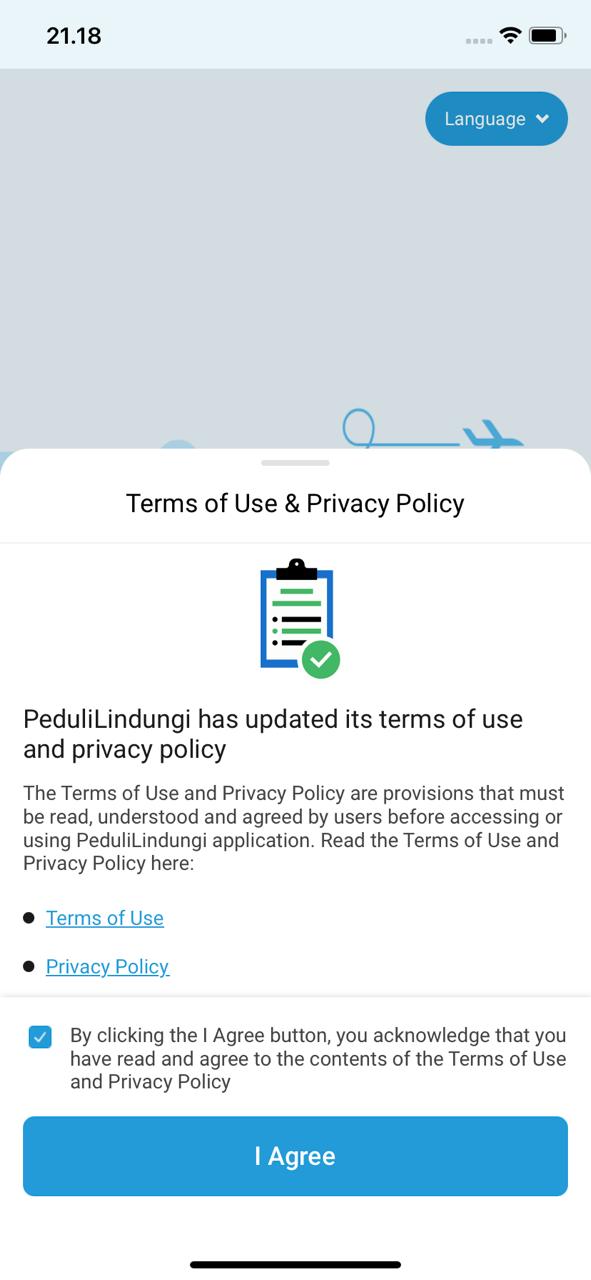The screenshot image displays a user privacy agreement prompt from the Peduli Linguae application.

**Header Section:**
- The top of the screen has a light blue background featuring the time "21:18" on the left side.
- On the right side, there are four horizontal dots, a Wi-Fi symbol, and a battery icon.

**Mid-Section:**
- Directly beneath the top bar, there is a gray background strip on the right side with a language selection option highlighted in blue. This strip takes up the top third of the image.

**Main Content:**
- Below the gray strip, terms of use and privacy policy details are displayed prominently. 
- There is a crucial notification stating that "Peduli Linguae has updated its Terms of Use and Privacy policy," followed by detailed provisions specifying that users must read, understand, and agree to these terms before accessing or using the application.
- A call-to-action line, "Read the terms and use of the privacy policy here," is shown with "Terms of Use" and "Privacy policy" written in blue text, which are clickable links.

**Footer:**
- At the bottom, there is a checkbox that is already checked beside the text, "Please click and agree button."
- Directly below this, the user is prompted to proceed with an "I agree" button highlighted in blue.